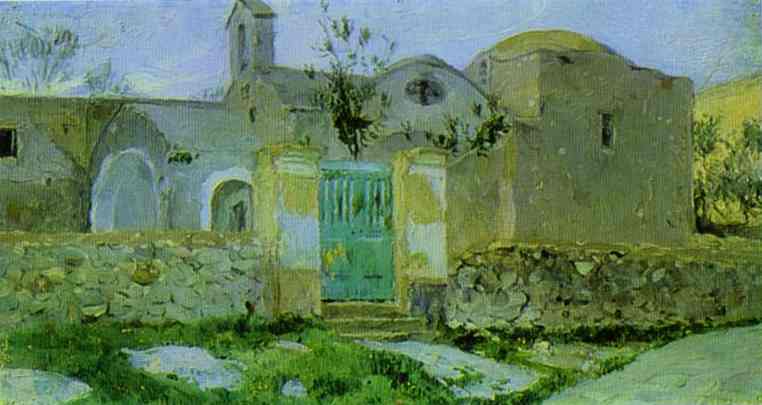The painting depicts a vintage Spanish-style stucco house, possibly a church, characterized by its distinct architectural features. The structure includes a dome-shaped steeple or bell tower on the roof, suggesting a religious function. The building, set against a backdrop of a blue sky with scattered white clouds, is primarily depicted in shades of green and blue. 

The white church-like building is bordered by a low grey stone wall interwoven with a green fence, blending seamlessly into the surrounding landscape. The entrance features French doors opening to the side, accompanied by three steps leading up to them. There are a few small windows scattered around the façade, enhancing its antique charm. 

To the right of the building, a flat grey road runs by, while a yellow sloping hill adorned with various green trees rises in the background. The painting’s lower portion is punctuated by patches of greenery and grass, adding to the serene, idyllic setting captured by the artist. Although the artist's name is not visible and might be cropped off, the detailed and somewhat blurry style imbues the scene with a nostalgic, almost dreamlike quality.